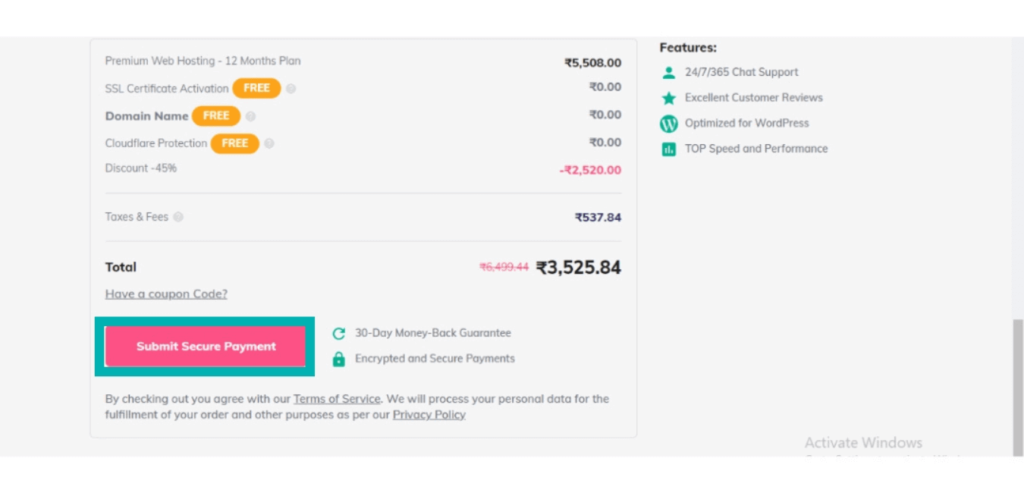**Website Screenshot Description:**

The image is a screenshot of a webpage with a gray background. On the far right, at the bottom, there's a dark gray vertical slider bar. In the bottom right corner, a watermark reads "Activate Windows."

The page lacks a header. Towards the left side, a box contains various pieces of information primarily written in light gray or black text. From the top, the content reads:

- **Premium Web Hosting 12-month plan:** The price listed is 550800, though the currency symbol is unclear.
- **SSL Certificate Activation:** Accompanied by an orange button labeled "Free" with a zero cost.
- **Domain Name:** Boldly displayed with a free orange button next to it, indicating zero cost.
- **CloudFlare Protection:** Marked as free with a yellow-orange button, also indicating zero cost.

A discount is noted as "-45%", translating to a total reduction of 2,520 in red. 

- **Fees and Taxes:** Listed as 537.84.
- **Total Cost:** Initially displayed as 5,400 or 6,499.44 in red with a strikethrough. The final total, highlighted in bold black, is 3525.84.
- **Coupon Code:** A prompt for entering a coupon code.

Below the total cost, there is a green button with a red square, containing the text "Secure Payment" in white letters. 

Additional information includes a "30-day money-back guarantee," encrypted and secure payments notice, and a message confirming that by checking out, users agree to the terms of service and the processing of personal data according to the privacy policy.

On the right side, at the top, in black text, the section titled "Features" is outlined with four green symbols stating:
1. 24/7, 365 chat support
2. Excellent customer reviews
3. Optimized for WordPress
4. Top speed and performance